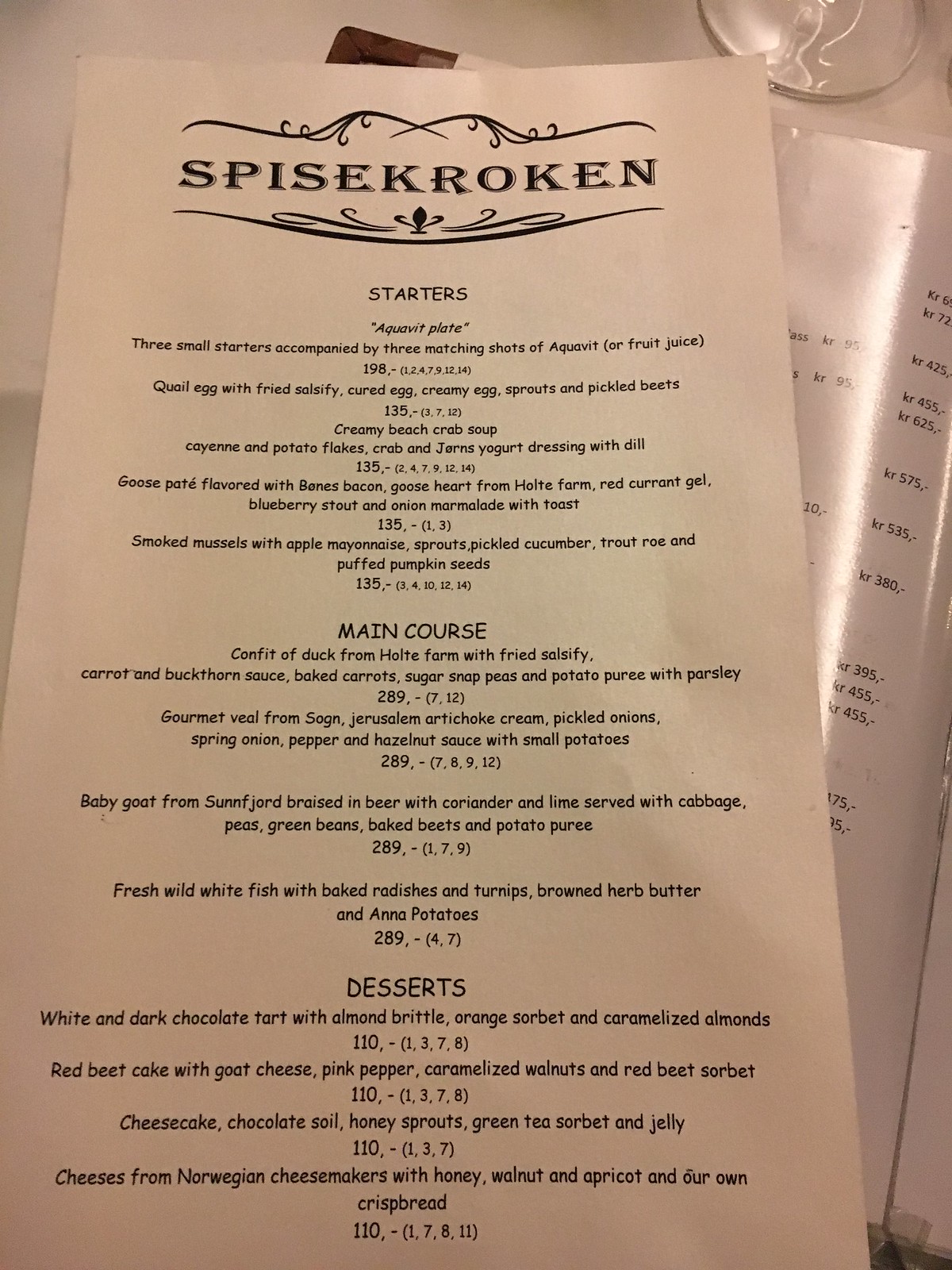Top-tier dining experience menu overview:

**Brand Name: [Brand Name]**

**Starters:**
- **Aquavit Plates:** A selection of three small starters, each paired with a matching shot of Aquavit or fruit shoots.
    - **First Plate:** Quail egg with fried salsify, cured egg, creamy egg sprouts, and pickled beets.
    - **Second Plate:** Creamy beach crab soup.
    - **Third Plate:** Goose pate flavored with bacon-boned goose heart from Hody Farm, accompanied by red currant gel, blueberry stout, and onion marmalade on toast.
- **Smoked Mussels:** Served with apple mayonnaise.

**Main Courses:**
- **Duck Confit:** Sourced from Holtz Farm, served with fried salsify.
- **Gourmet Veal:** Hailing from Soggin, featuring Jerusalem artichoke cream and pickled onions.
- **Baby Goat:** Sourced from Sunfjord, braised in beer with coriander and lime, and served with cabbage.
- **Fresh Wild Whitefish:** Accompanied by baked radishes and turnips, served with browned herb butter.

**Desserts:**
- **White and Dark Chocolate Tart:** Topped with almond brittle.
- **Red Beet Cake:** Paired with goat cheese.
- **Classic Cheesecake**
- **Cheese Selection:** A variety of cheeses from Norwegian cheesemakers, served with honey.

**Note:** This menu showcases an exquisite array of starters, main courses, and desserts, highlighting the use of fresh and locally-sourced ingredients.